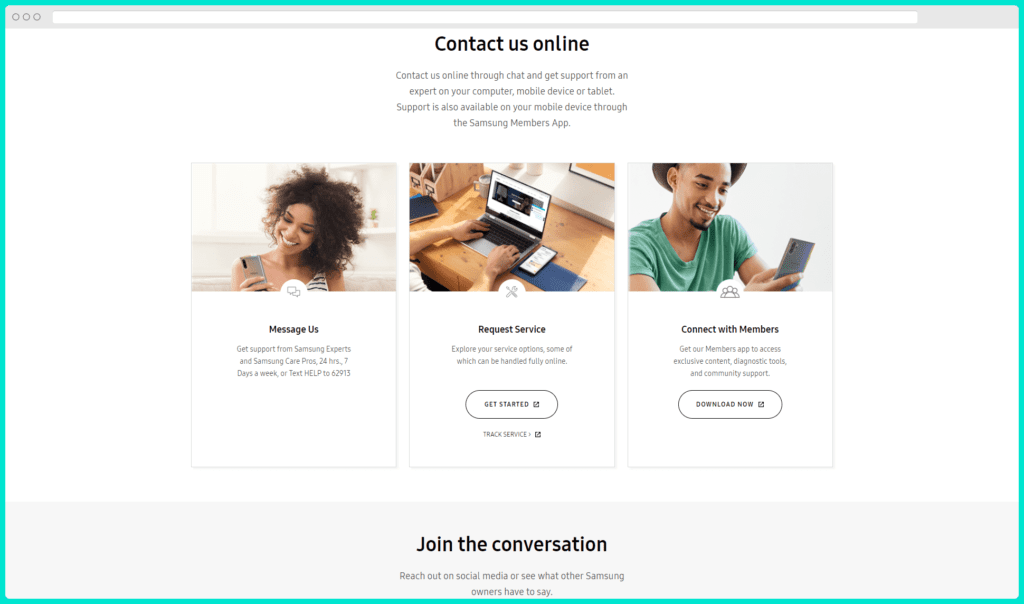This is a screenshot of a speculative website design. At the top of the image, there is a gray bar that features an empty white field where the web address would typically appear, suggesting the site is a mockup rather than a functional website. Below the gray bar, the background is white with black text that prominently reads "Contact Us Online." In smaller black font beneath this heading, the text elaborates: "Contact us online through chat and get support from an expert on your computer, mobile device, or tablet. Support in this is also available on your mobile device through the Samsung Members app."

Further down the page, there are three horizontal advertisement-style photographs that appear to be stock images. 

1. On the left, there is an image of a smiling Black woman with fluffy afro hair, looking at her phone in a minimalist, pure white kitchen.
2. In the center, there is a close-up photo of a person's hands typing on a laptop keyboard.
3. On the right, there is a Black man wearing a fedora and a gray t-shirt. He has a mustache and goatee and is holding a phone while smiling.

These images collectively emphasize the availability and accessibility of online support across various devices and settings.